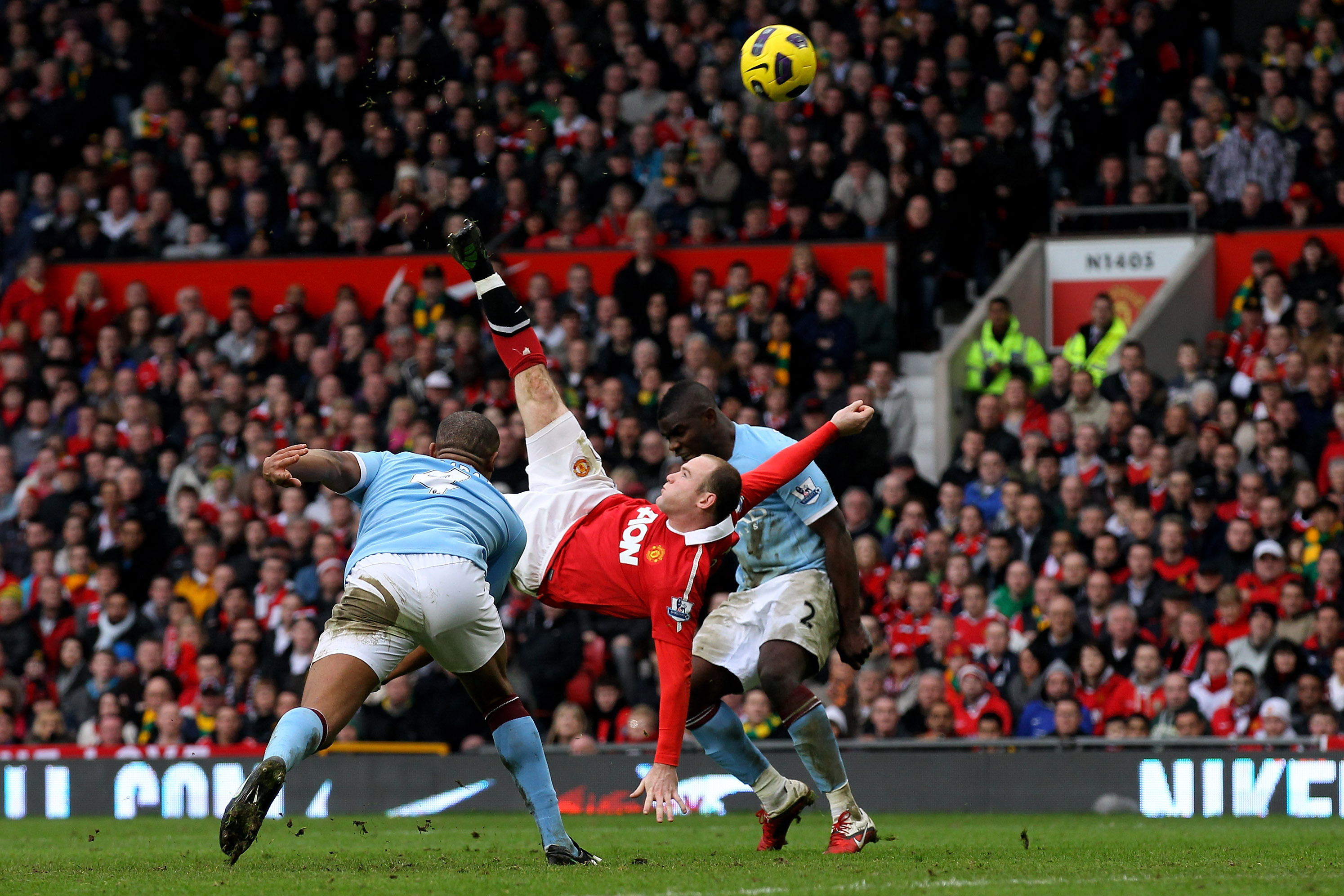In this detailed image capturing an intense moment of a soccer game, a player in mid-air, wearing a red jersey with white shorts, executes a flip kick aiming at a yellow and black soccer ball. This Caucasian player, centrally positioned in the action shot, is flanked by two African players from the opposing teams, both dressed in light blue jerseys, white shorts, and long light blue socks. The background reveals a packed stadium filled with blurry heads of cheering fans, emphasizing the game's high energy and large attendance. Visible above the vibrant green field is a long gray banner bearing the iconic white Nike logo and additional advertisements. Brightly visible near one of the levels' entrances, two security personnel in reflective yellow vests stand guard, further accentuating the lively but orderly atmosphere of this soccer match.